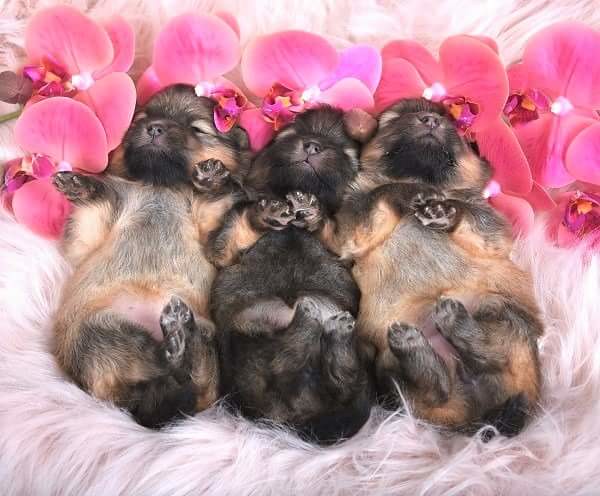In this professional studio photograph, three adorable puppy dogs are lying on their backs, nestled together on a plush, white, shaggy cushion. The puppies, appearing to be the same breed, are all fast asleep with their eyes closed and tiny paws in various positions – the two on the right having their paws together while the one on the left has its paws spread out. Their soft bellies are exposed, showcasing a mix of light and darker fur, with the middle puppy predominantly black in contrast to the lighter hues of the ones on each side. Above their heads, delicate pink orchid-like flower petals, resembling plumerias, add a charming touch to the serene scene. The well-lit setting, devoid of any text or artist signature, focuses solely on the innocent tranquility of the sleeping puppies, creating an irresistibly cute and heartwarming image.